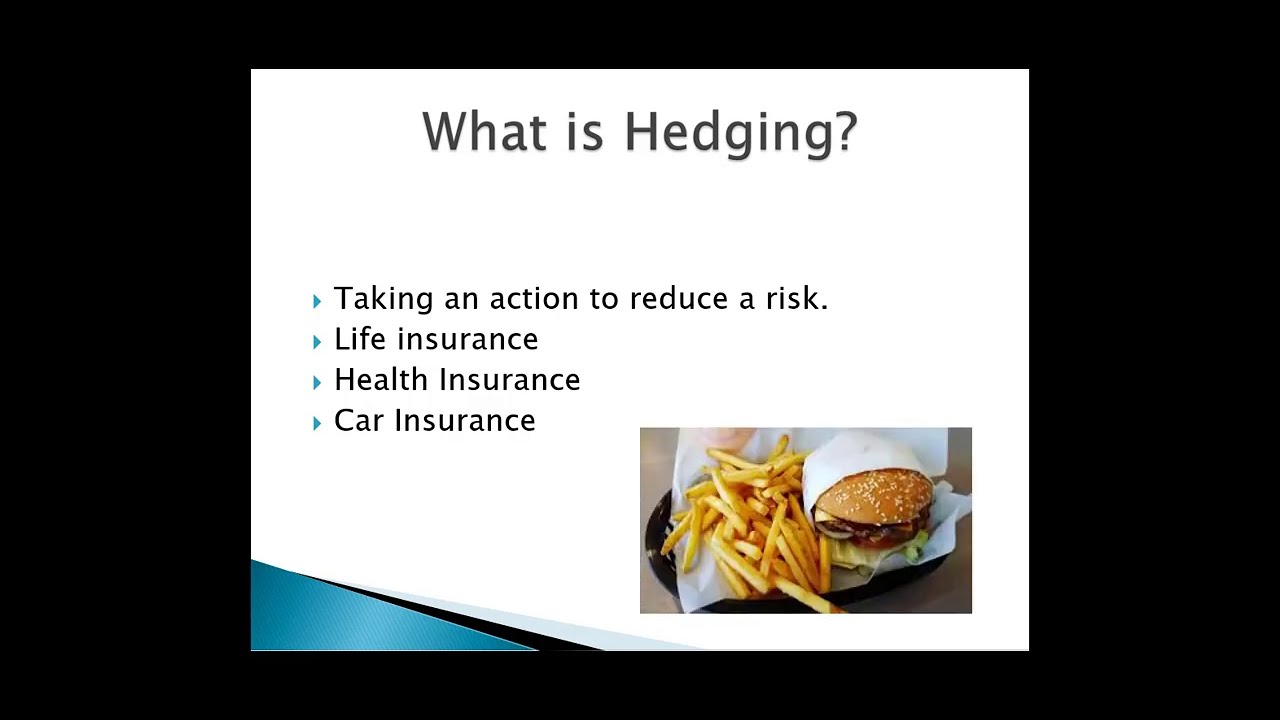This image appears to be an advertisement or educational slide explaining the concept of hedging in a detailed manner. It is designed as a rectangular horizontal image with a black background, inside which there is a smaller white rectangle. This white rectangle features a bold title at the top in large black letters that reads "What is Hedging?" Directly below the title, in smaller black letters, are four bullet points, each marked with blue triangle bullets. The bullet points explain hedging as "taking an action to reduce a risk" and provide examples like "life insurance," "health insurance," and "car insurance." Additionally, the top left corner of the white slide has a lighter blue diagonal accent. In the bottom right corner, unexpectedly, there is an image of a hamburger partially wrapped in butcher paper accompanied by a pile of French fries. The very corner of the white rectangle is also slightly lifted on the left side, revealing some blue underneath, adding a subtle design element to the layout.